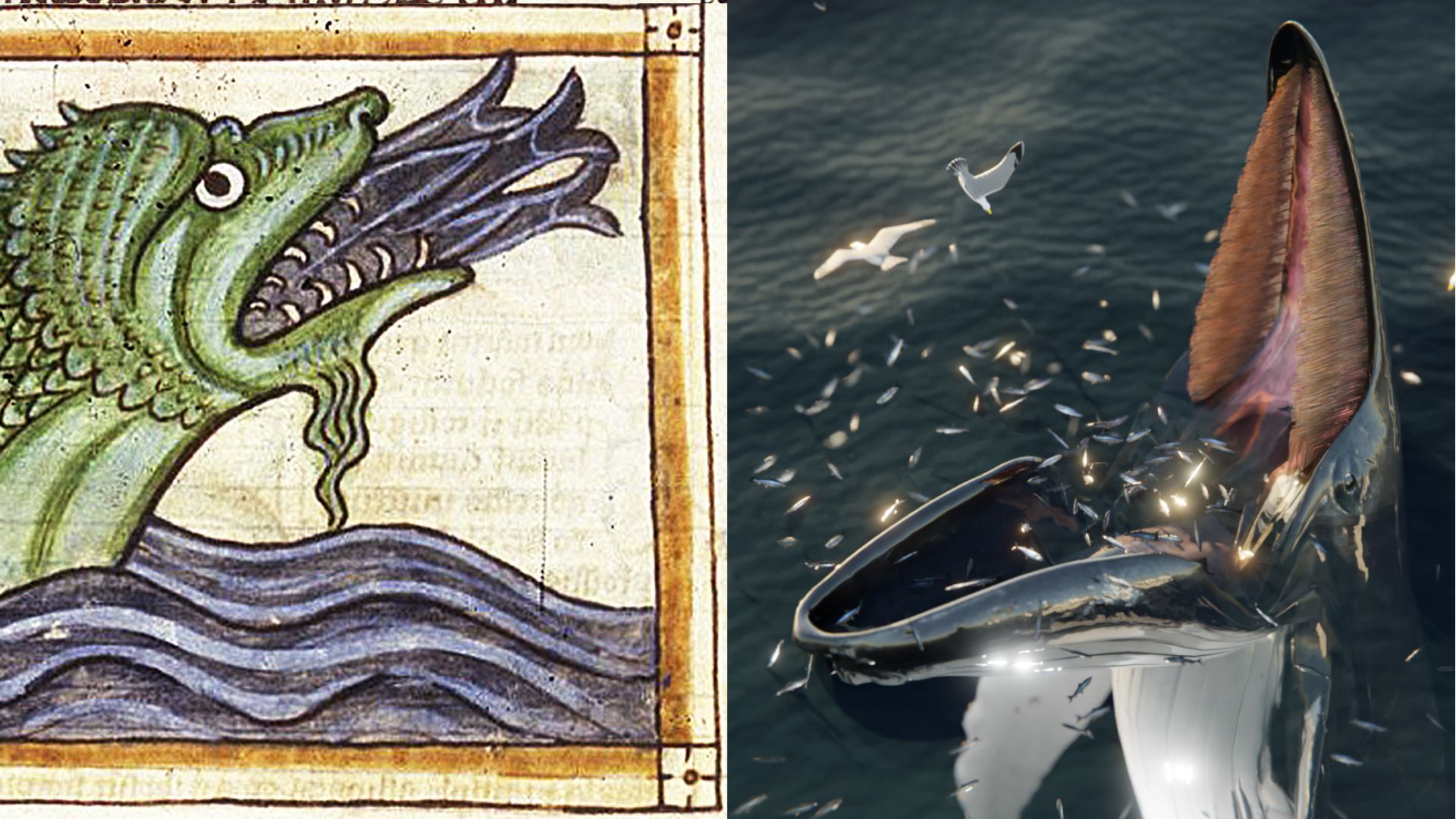The image consists of two side-by-side pictures of equal size. The left picture is a colored drawing featuring a green sea monster with a scaly, pointy head and a beard. This sea creature, with sharp-edged teeth and a forked tongue, is emerging from blue and purple waves that reach up to its neck. The monster has several fish in its mouth and the artwork is framed on the top and right side with brown coloring, suggesting it was created with crayons or paint. 

The right picture resembles a photograph but clearly has been digitally manipulated. It depicts an enormous sea creature or possibly a sea mammal in open water, with a mouth gaping open at nearly a 90-degree angle. The top of its mouth is pink while the bottom part is black, and the inside is filled with brightly lit fish. The creature’s head is partially black with some white underneath its mouth, and fins are visible. In the surrounding water, numerous fish can be seen, and there are two white birds—one flying and one standing on the water—near the creature. This image has been constructed using computer imaging techniques.

Together, these pictures contrast a mythical sea monster with an exaggerated sea creature captured in a realistically styled yet digitally altered photograph, both depicting scenes of feeding amidst the waves.